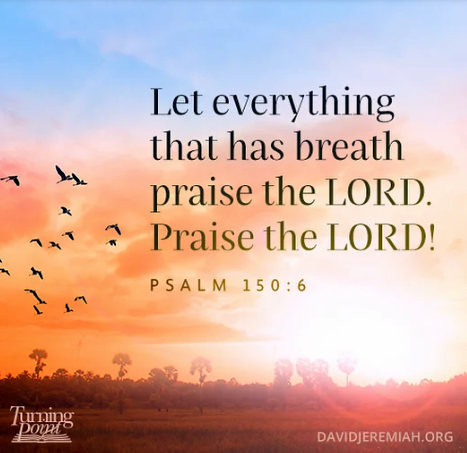This image, perfectly square in shape, resembles something typically posted on Facebook. It captures a serene scene of birds flying across a sky transitioning from deep blue at the top to a warm orange near the horizon, suggestive of either a sunrise or sunset, over what appears to be the savannah. The sunlight bathes the distant trees and ground in a reddish-green hue, adding to the natural beauty of the setting.

Central to the image is an inspirational message in black text that reads: “Let everything that has breath praise the Lord. Praise the Lord.” The second "Praise the Lord" is emphasized with an exclamation mark, and the scripture reference “Psalm 150:6” is noted below in brown. In the corners of the image are additional textual elements: in the lower right, in white text, is the website “DavidJeremiah.org” and in the lower left, also in white, is the "Turning Point" logo designed to resemble an open book made of simple white strokes.

This beautifully crafted image, blending an evocative natural landscape with a powerful spiritual message, aims to inspire and uplift.